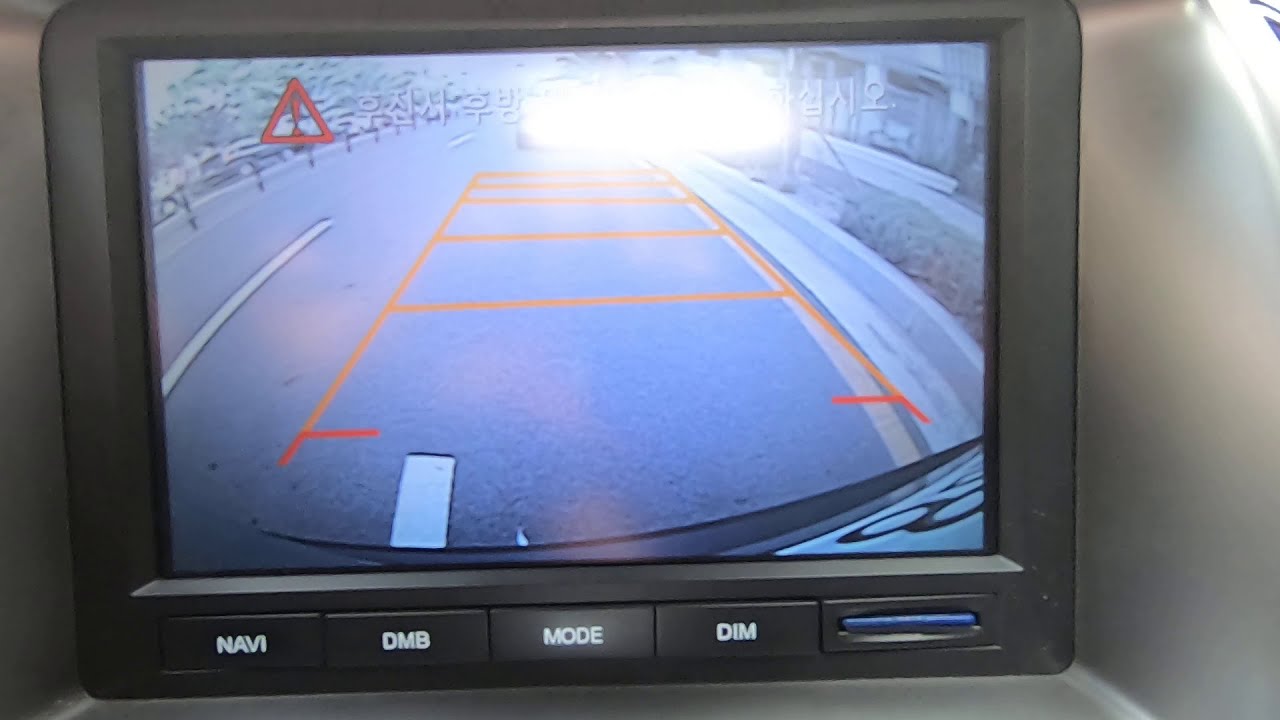The image displays a surveillance-like backup camera screen inside a vehicle, showing parking alignment guidance with orange lines indicating the car is not properly aligned with the parking spot. The screen is bordered by a black frame and includes a detailed view of a road with curbs on both sides and some grass on the right-hand side. Prominent Asian, likely Chinese, lettering appears on the upper right corner, while a red caution triangle with an exclamation mark is visible in the upper left corner. At the bottom of the screen, there are various buttons labeled "Navi," "DMB," "Mode," and "DIMM," and an SD card slot to the right. The overall display is set within what appears to be a white plastic dashboard, with a small glare on the screen.